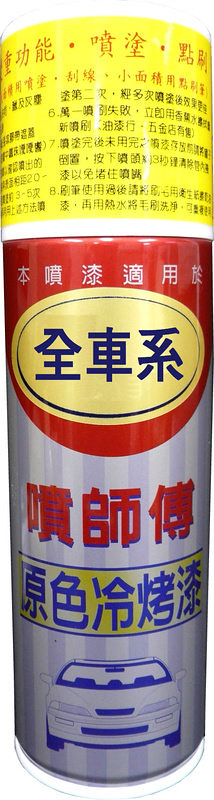The image depicts a product in an aerosol can placed against a white background. The can features a bright yellow lid, transitioning into a red section adorned with black and red foreign characters, likely Chinese or Japanese. Just below this, a prominent golden oval contains blue text. The can then tapers into a silver section, which includes additional red writing, followed by a yellow banner with more blue characters. Finally, at the bottom of the can, there's a detailed illustration of a white car. The design elements and labeling suggest it could be a car-related product, possibly wax or spray paint.